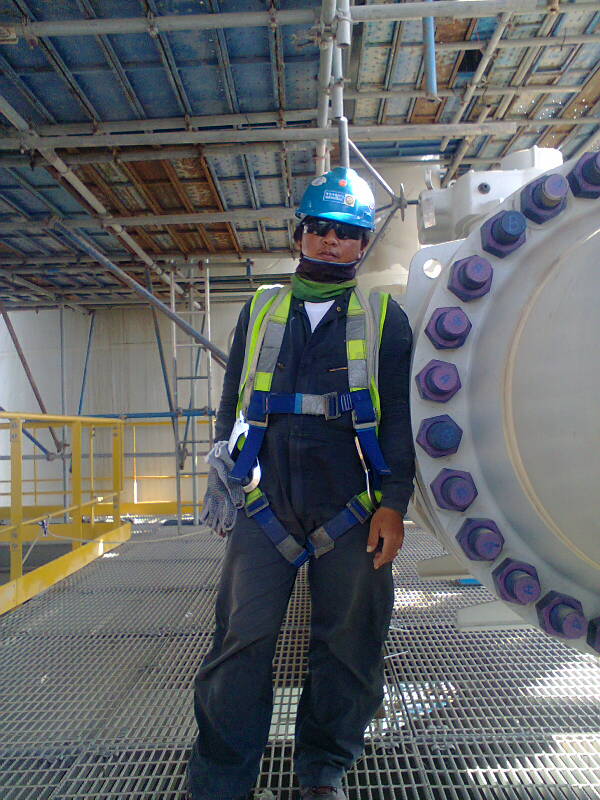The image depicts a worker, likely an engineer or construction/factory worker, standing on a large, rectangular, gray metal grate floor situated high up in an industrial building. The floor allows visibility to the area beneath due to the grate design. To the worker's left and right, yellow safety railings are visible, providing support and preventing falls. The backdrop features an unfinished ceiling with corrugated metal panels and visible insulation, indicative of factory settings.

The worker is dressed in a blue, long-sleeved, long-legged boiler suit reminiscent of traditional workwear, resembling a one-piece jumpsuit. Over this jumpsuit, he dons a high-visibility safety vest, striking in a bright yellow color. Further adding to his safety gear, he wears a blue hard hat and a pair of dark sunglasses. Around his neck, a piece of fabric is wrapped, possibly for additional warmth or protection. His attire also includes straps around his legs and chest, hinting at an integrated safety harness system, and in his left hand, he holds work gloves.

Beside him, on his right, stands a large cylindrical object. This object is a section of white piping, bolted together with very large, colorful bolts—blue or purple in some mentions. This massive pipe is significantly larger than the worker’s body in width, underscoring its industrial scale and utility.